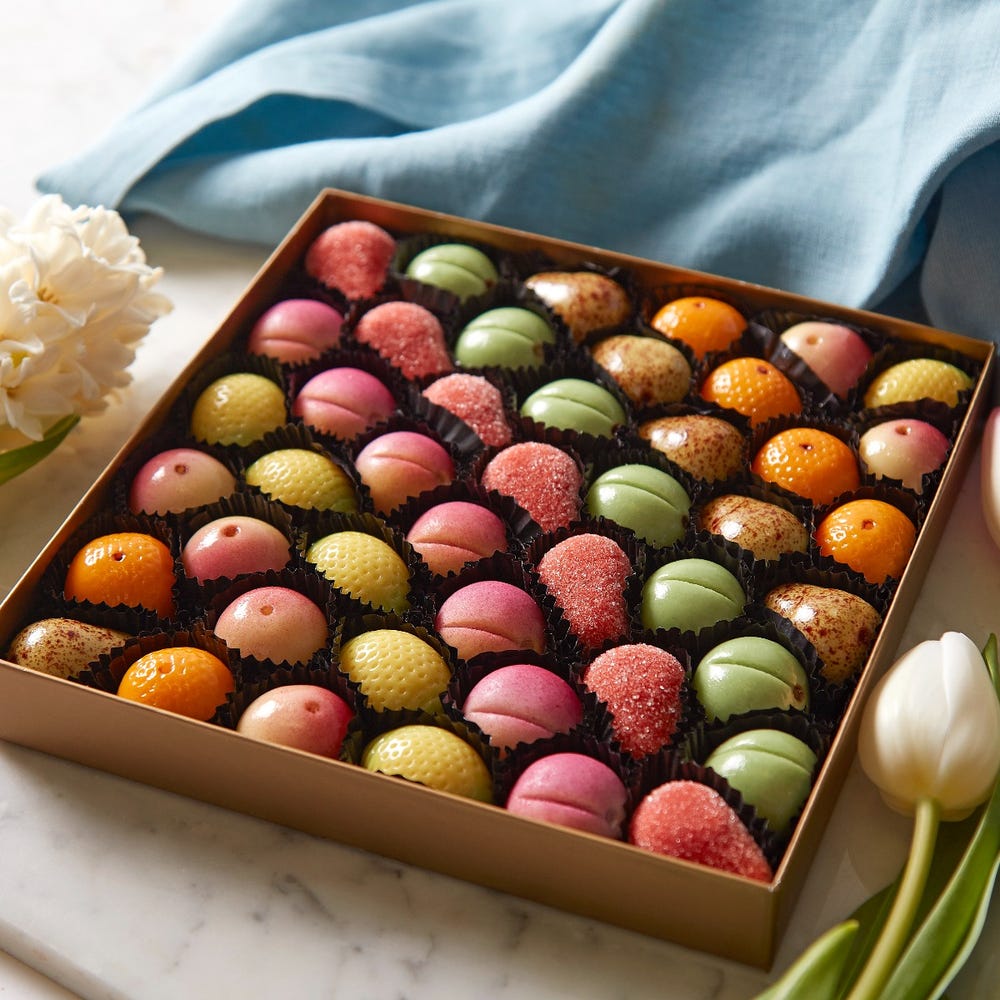This image showcases a golden box of intricately crafted marzipan shaped like various fruits, each nestled in individual brown paper wrappers. The vibrant marzipan fruits include oranges, peaches, lemons, strawberries, pears, and others, arranged diagonally within the box. The box rests on a white marble surface adorned with a single white tulip to the bottom right and a bundle of fluffy white flowers to the left. A soft, blue cloth is gently laid out behind the box, adding a touch of elegance to the scene. The marzipan is detailed with different textures and colors, such as orange speckled pieces, yellow sections with small indents, pink and white varieties, green pistachio-colored ones, and red sugar-coated pieces, giving the assortment a rich, gourmet appearance.